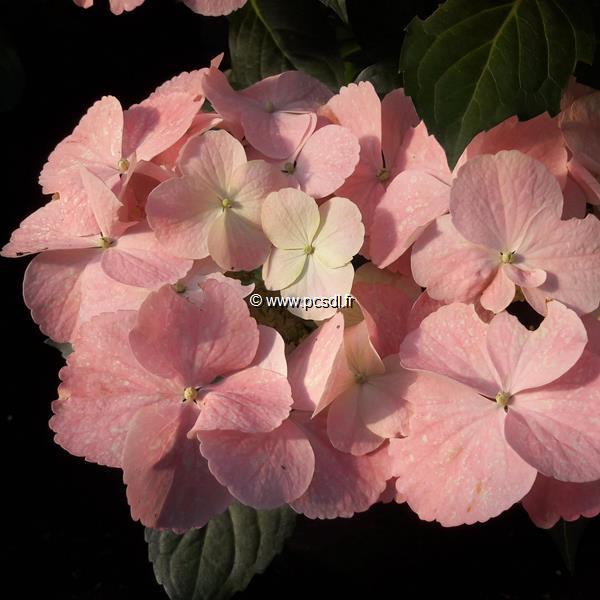The image showcases a cluster of pink flowers, each with circular, light pink petals that faintly blend into white hues. The flowers are thin and flattened, layered upon one another, and are illuminated by bright sunlight which casts a warm glow over them. Each bloom features a small yellow stamen at its center and is surrounded by large, faded green leaves, both in the foreground and as part of the background. The overall backdrop of the image is dark, creating a striking contrast with the vivid, sunlit flora. In the center of the image, white text that reads "© www.pcsdl.fr" is overlaid, indicating it is hosted on a French website. Some flowers are cut off at the top left, contributing to the organic, clustered appearance.